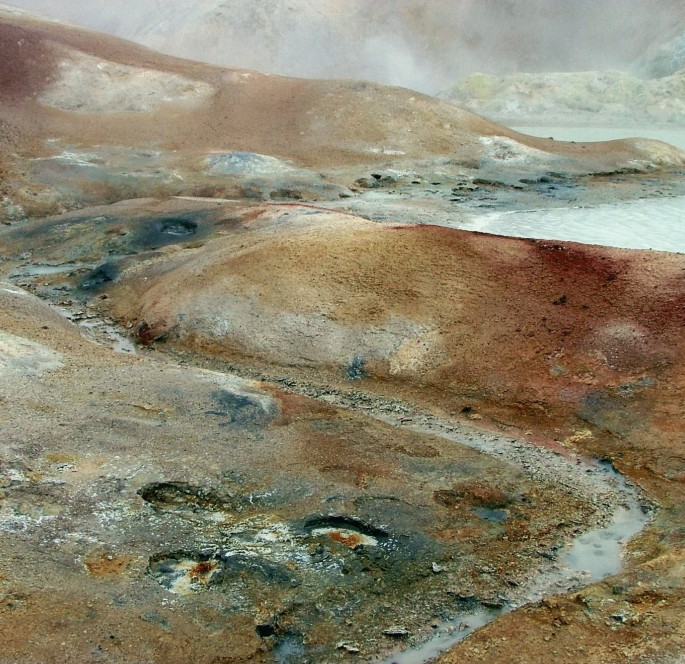The image depicts a desolate and eroded landscape, resembling a watercolor painting of a beach area. The scene features various shades of sand, including brown, red, blue, and white, indicative of diverse mineral deposits interspersed with small rocks and pebbles. This sandy expanse forms gentle hills and mounds, some eroded to the point of displaying linear stream or river channels carved into the earth. Warm, calm waters from a nearby cove flow into these channels, creating pools and depressions that may be tinged with pollutants. The landscape extends into the background with larger water pools and possibly limestone formations shrouded in a misty atmosphere, adding to the sense of distance and isolation. Above, a dark, stormy sky looms, filling the scene with a sense of foreboding and emphasizing the area’s rugged and eroded state. The overall impression is one of natural but damaged beauty, with the landscape showing scars of environmental wear and possible pollution.